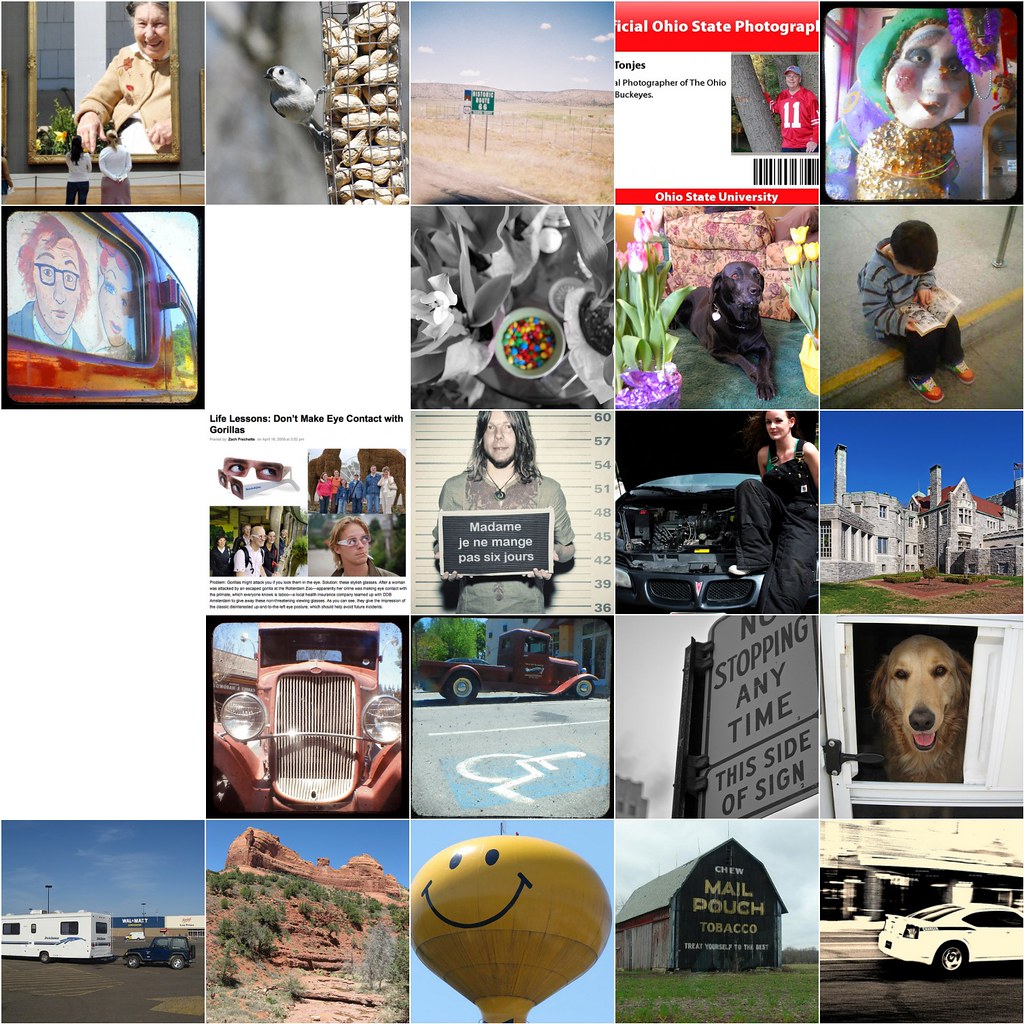The image is a 5x5 grid of 25 different square photos, each offering a unique glimpse into various scenes. Notable among these are a yellow water tower with a smiley face located in the bottom middle, and just to its right, a barn featuring the text "Mail Pouch Tobacco." In the fourth row on the far right, a golden retriever is seen peeking through an open door. Centrally positioned, a man with long brown hair holds a black board inscribed with French words, reminiscent of a mug shot. The third and fourth rows on the left have entirely blank white squares. Additional images include a lady peering out a window, two individuals observing a large framed photo, a desert landscape, a mysterious doll, black and white photos, another dog, a yellow balloon with a smiling face, a farmhouse, an RV camp, mountains, and various candid shots of people and animals in different settings.